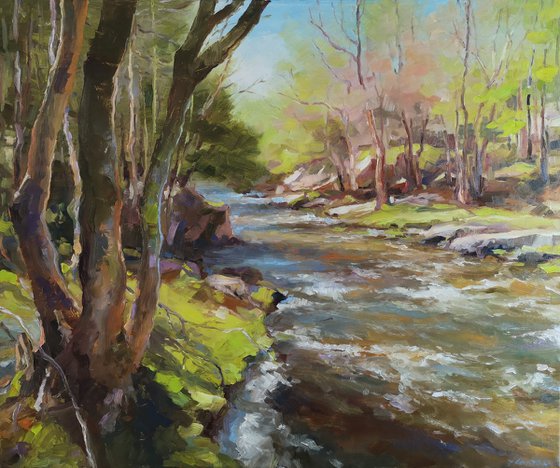This square canvas painting, likely done in a painterly, impressionist style perhaps using oil paints, vividly captures a serene natural scene with a flowing creek. Stretching from the bottom right towards the background, the creek starts with a brown hue at its base and transitions to rippling white waves and a bluish tint further back. Surrounding the creek are rocky riverbanks adorned with slate-like stones and grassy areas. On the right side of the painting, the terrain is rocky and hilly, populated by trees bearing a mix of green and red leaves, some of which are bare. Towards the upper right, the blue sky is subtly visible. 

The left side of the painting features a prominent tall tree with multiple limbs and a mix of light and dark brown shades, set against a backdrop of green grass. Surrounding this tree are other green trees and some with highlighted white trunks, providing a sense of depth. The vibrant foliage varies from greens to an array of pinkish hues, adding to the dynamic and colorful depiction of nature. Birds can be seen flying against the blue sky, adding to the serene and picturesque quality of this detailed and textured landscape.